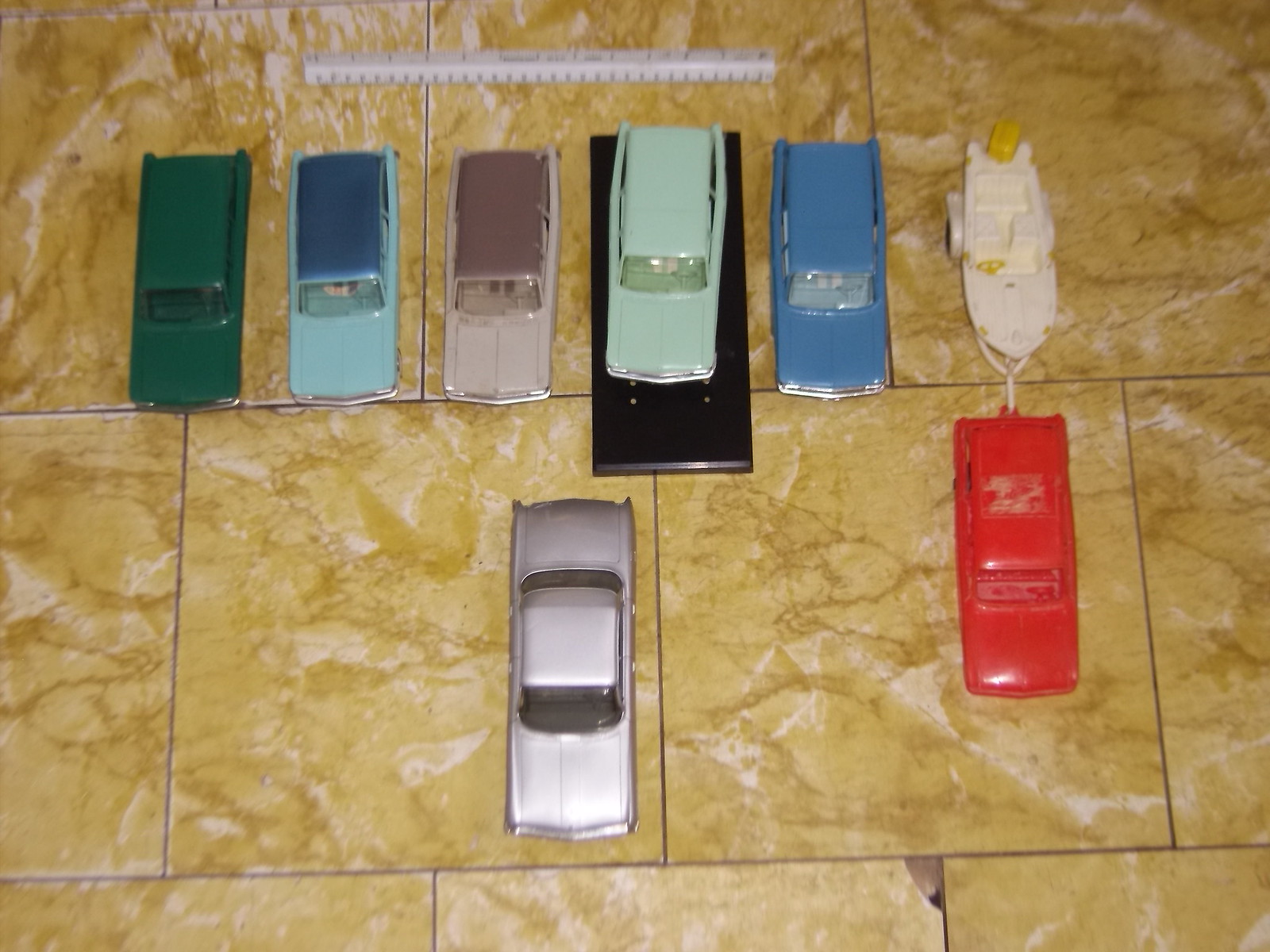The image depicts an older, pixelated, and slightly blurry photo taken indoors, showcasing a collection of toy vehicles displayed on a dated, ugly, and chipped tiled countertop, which has a yellowy-orange to brown swirl pattern. The countertop features thin gray grout between the tiles, one of which is chipped at the upper corner revealing gray underneath. There are a total of seven cars in various pastel colors and a white boat being towed by a red toy truck. Among these, the colors include blue, purple, green, and silvery-purple, with specific details like a green car, two gray cars with blue and green roofs respectively, a white car on a black holder, and a light blue car. Additionally, a ruler is placed at the top of the image, possibly to indicate the size of the toys, which appear to be around three inches wide.